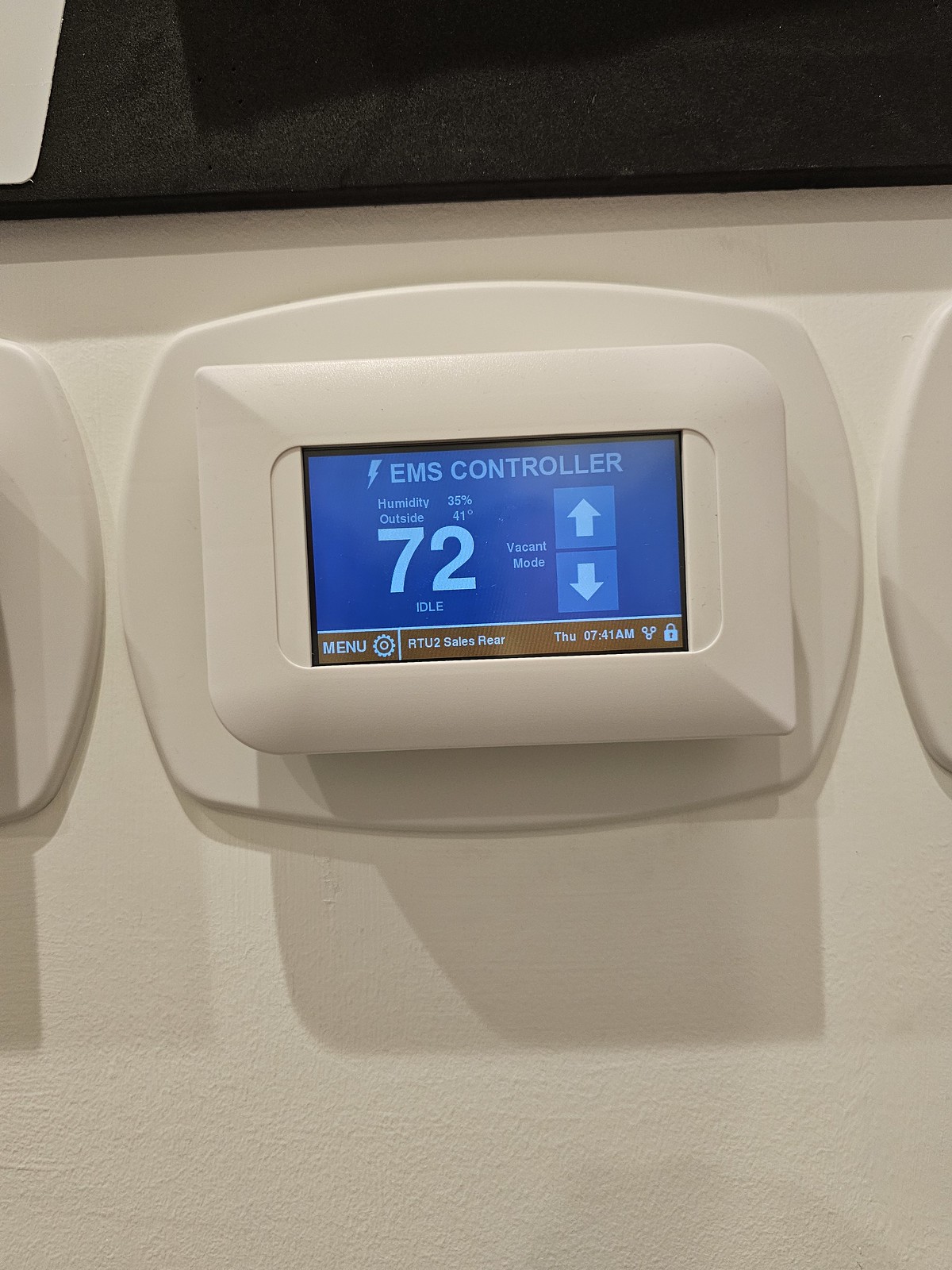The image features a white countertop with a whip in the background. Behind the whip, there is a black object, possibly an oven or a stovetop. On the countertop sits a two-piece plastic device. The top piece is a white rectangular box with slightly curved corners, housing a blue screen. The screen displays the text "EMS Controller" with a lightning bolt symbol preceding the 'E'. It also shows the number '72', along with upward and downward arrows. Below the arrows, there is a "Menu" option within a brown rectangular box at the bottom of the blue section. The lower part of the device is a wider rectangular plastic base.